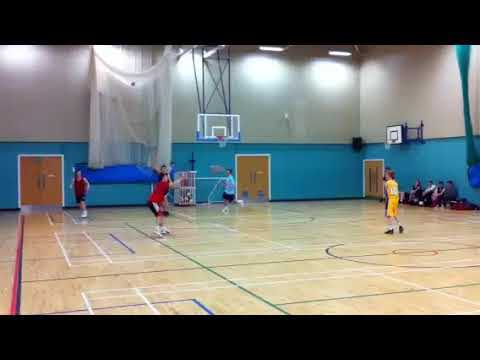This image captures an indoor basketball court scene, framed with a thick black border at the top and bottom. The gym's walls are a striking combination of white on the upper portion and blue on the lower, with three double doors embedded within the blue section. The gym is illuminated by bright fluorescent lights, with visible light fixtures hanging from the ceiling.

On the court, there are around five players engaged in play, with indistinct motion blur adding a dynamic sense of action. The floor of the court is a typical light brown tile, marked with black, white, and blue lines. One basketball hoop is prominently visible in the upper middle part of the picture, while another hoop appears on the right wall.

Several of the players are identifiable by their attire: two are wearing red jerseys and black shorts, one is in a blue T-shirt with dark shorts, and another stands out in a full yellow kit with a white number. To the right side of the image, a small group of four individuals is seated on the pale brown floor, leaning against the blue portion of the wall, enhancing the communal and relaxed atmosphere typical of a gym during practice or a casual game.